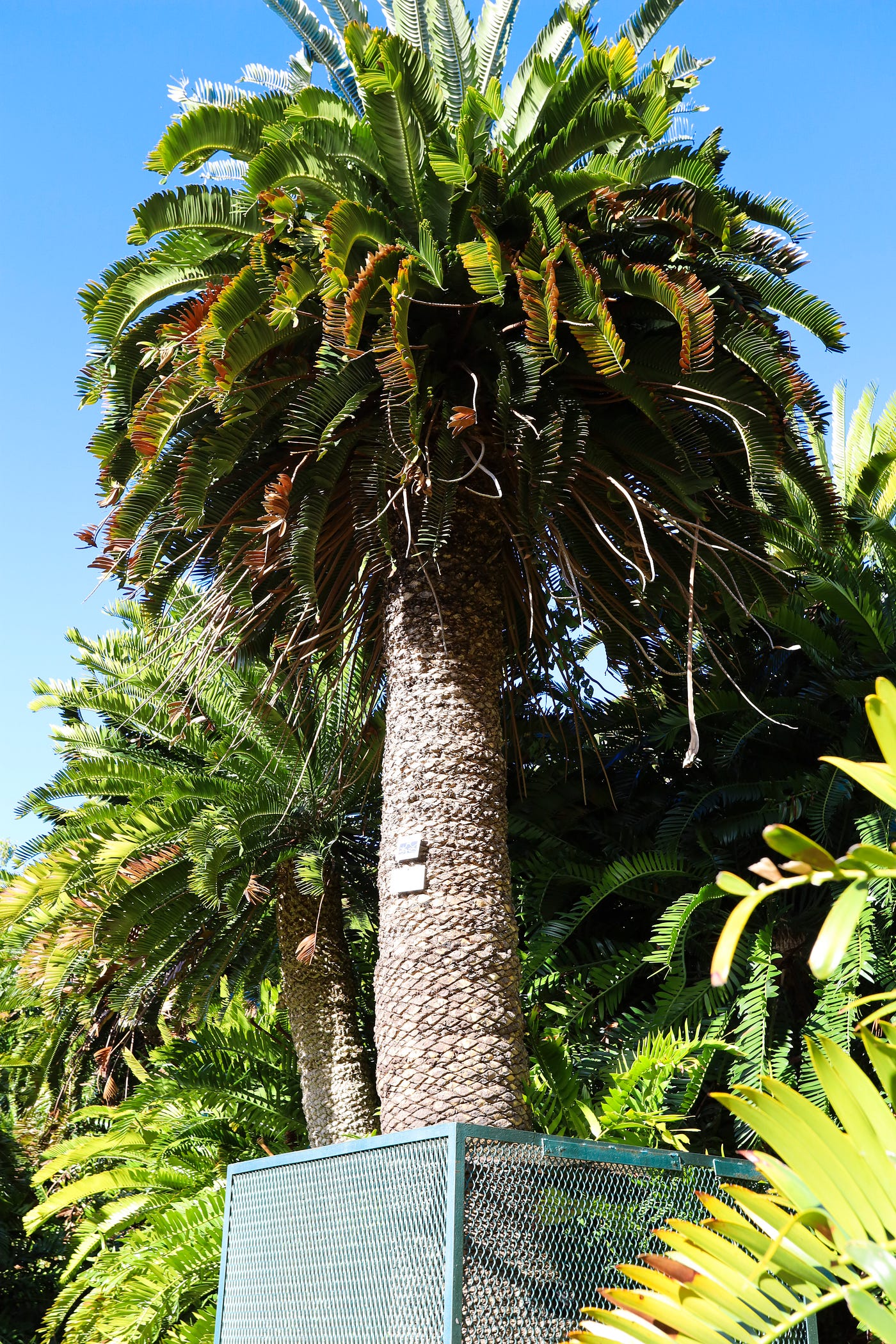The image captures a large, imposing palm tree that conspicuously stands out in the foreground. The tree, although resembling a natural palm, has unmistakable signs of being a disguised cell phone tower. At the top, thick fronds splay out in a lush, rounded formation, but closer inspection reveals suspicious metal components embedded in the trunk and a pair of man-made boxes attached midway up. The tree's base is encircled by a greenish metal cage, which hints at its artificial nature. Despite these odd features, the faux palm blends quite seamlessly into its surroundings, which include several other authentic, densely foliaged palm trees laden with fruit. The scene is bathed in bright sunlight under a vivid blue sky, entirely devoid of clouds, casting shadows that play across the verdant landscape. In the immediate foreground, fronds brush across the bottom right of the image, adding depth and a sense of proximity.